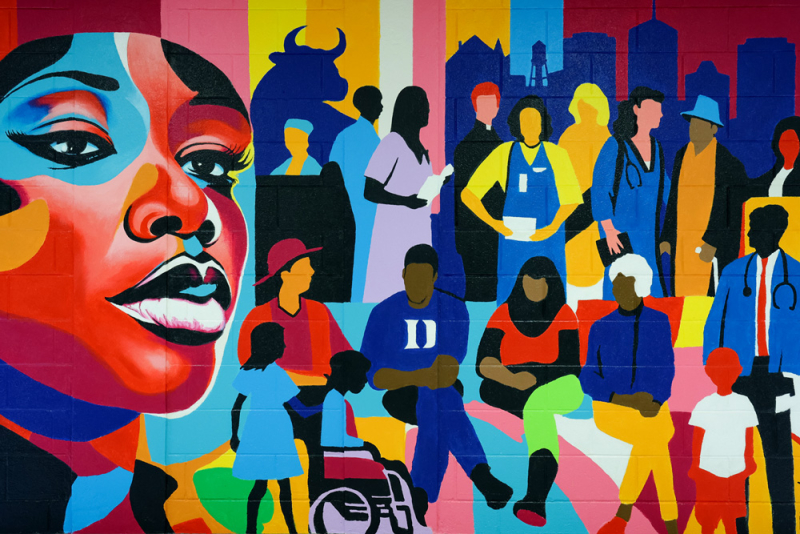This detailed mural, likely situated indoors, features a vibrant depiction of diversity and inclusion. The focal point on the left is a prominent face of an African-American woman, whose expressive features are accented with hues of blue and red. Her presence is a standout among the rich tapestry of colors that fill the mural, including stripes of brown, pink, yellow, and orange in the background. Below her, there's a gathering of various individuals: a total of eighteen, with nine seated in front and nine more behind them. These figures represent a range of races, genders, and professions, including medical personnel like doctors and nurses, as well as other common roles such as waiters. 

Among them, a notable figure wears a Duke shirt, suggesting a possible connection to Duke University. Additionally, a person in a wheelchair emphasizes the mural's theme of inclusivity. Behind this diverse assembly, there is a silhouette of a cityscape and a cow, suggesting a sense of unity between urban and rural elements. The blue silhouette of the cow sits harmoniously with the people, subtly conveying that everyone, regardless of differences, belongs together. Overall, this mural is a striking celebration of community and diversity depicted through vivid colors and expressive artistry.